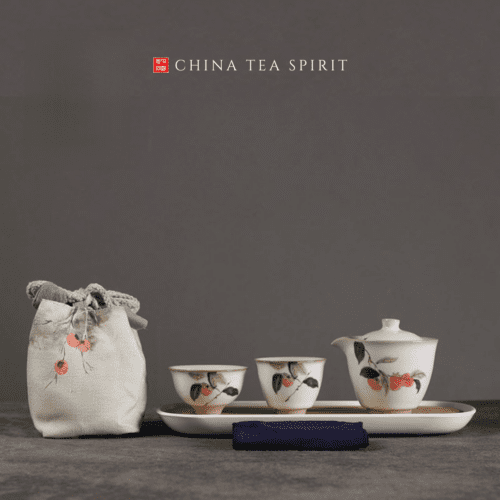This color photograph showcases a Chinese tea set displayed against a medium gray backdrop with a matching gray stone tabletop, which features subtle tones of light grayish-brown. At the top center of the image, small white lettering reads "China Tea Spirit" next to a quarter-inch red square logo with white Chinese characters. 

The tea set comprises a larger tea serving bowl and two teacups, all arranged neatly within a white serving tray. Each piece of the set, including the teapot with its lid, is adorned with a delicate floral print featuring dark green leaves and orange blossoms. The detailed floral pattern extends to a light gray, canvas-like sack positioned to the left of the tea set, which is likely used for storing tea leaves. 

Additionally, in the foreground of the image, there is a folded blue napkin, adding a touch of contrasting color. The overall composition of the photograph emphasizes the elegant design of the tea set, highlighting its intricate floral motifs and the brand's sophisticated presentation.